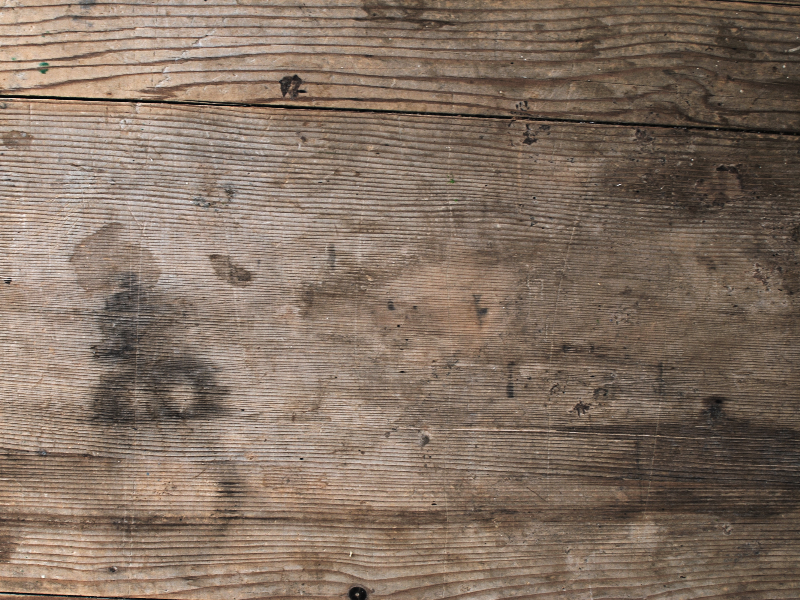This is a detailed and textured close-up photograph of an older, weathered piece of wood, taking up the entire frame. The wood surface is richly detailed with a variety of wood grains, colors, and notable marks. Predominantly light to medium brown, the wood exhibits darker brown rings, age lines, and patches of discoloration, indicating its age. There's significant wear and tear, noticeable through the many scratches, indentations, and an uneven, dirty appearance. The photograph reveals irregular black splotches, particularly on the bottom left and top right corners. A diagonal crack runs from the upper left to about three-quarters up on the right side. The left side of the image is brighter, suggesting the lighting source is from that direction. Additionally, there are gray discolorations, possible paint spills, and knots, with one knot prominently just left of center at the bottom, all adding to the complex character of the wood.